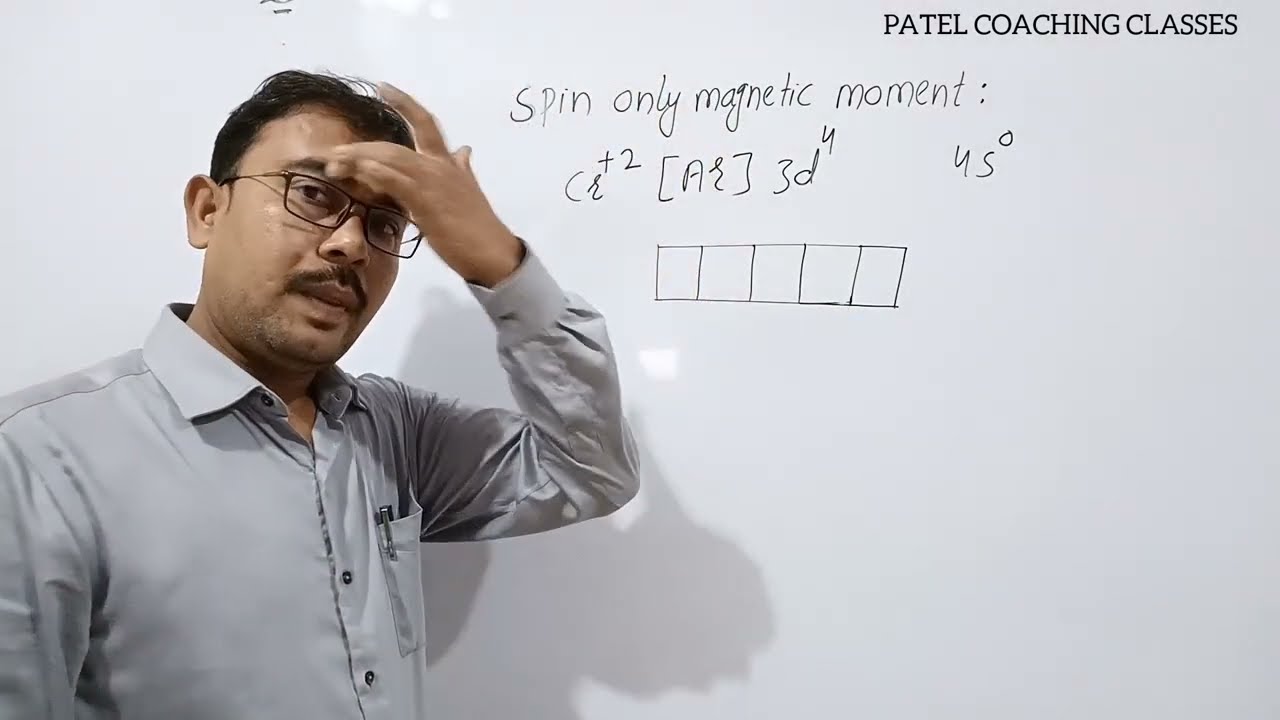In this image, a man, who appears to be a teacher, is deeply engaged in a lesson, most likely related to mathematics or physics. He is standing in front of a whiteboard, which prominently displays the handwritten phrase "spin only magnetic moment," accompanied by a complex math formula and a diagram featuring five squares arranged to form a rectangle. The upper right corner of the whiteboard features the text "Patel Coaching Classes" in bold, black, uppercase letters, indicating this might be part of a tutoring session or an online educational presentation.

The teacher, presumably Mr. Patel, is captured in a thoughtful pose with his left hand raised to his forehead, possibly pondering the next step in his lesson. His attire consists of a long-sleeve gray polo shirt with black buttons and a pen visible in the pocket, adding to his professional appearance. He has a darker brown complexion, dark brown hair, a mustache, and is wearing black-rimmed glasses. The scene is well-lit, casting a shadow of him on the whiteboard, enhancing the clarity and focus on his instructional stance.